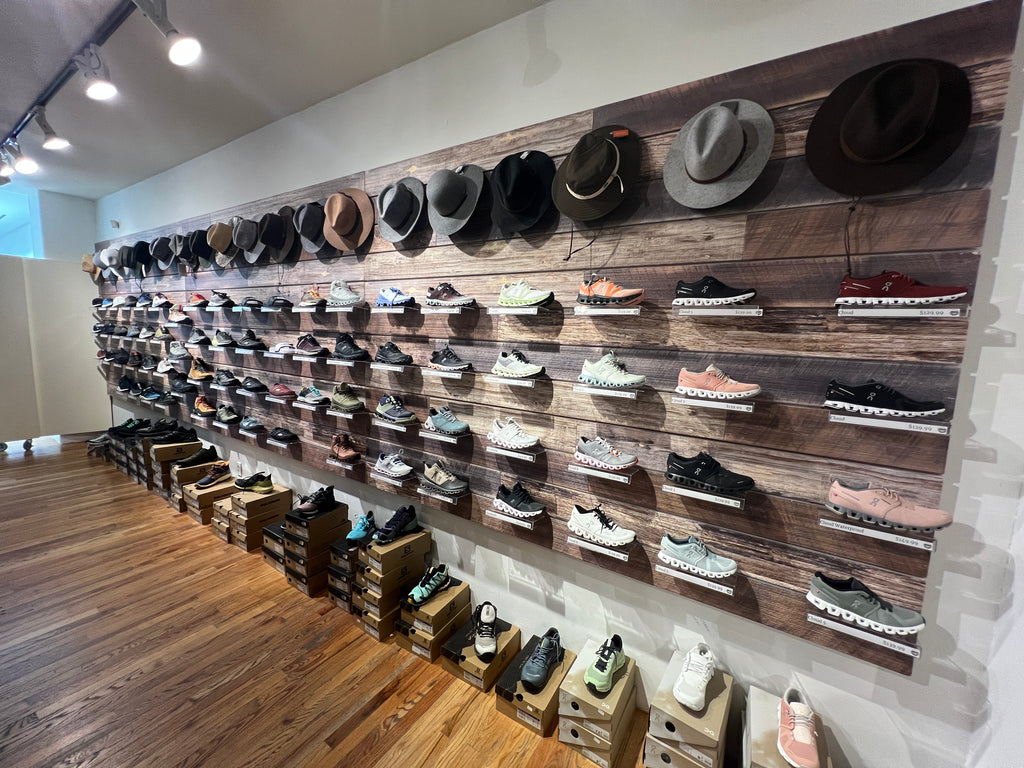The image depicts the interior of a specialty store prominently featuring sneakers and hats. The focal point is a wall in the center and right-hand side of the image, designed with wood board slats of varying shades of brown, gray, and tan, arranged both vertically and horizontally. This wall includes four floating shelves, each displaying a single sneaker on small protruding stands. Below these shelves, on a wooden floor, are stacks of shoe boxes, each topped with a corresponding shoe. The shoe boxes vary in number per stack, and there is no discernible pattern. Directly above the sneakers, a row of brimmed hats, likely made of leather or felt, is displayed on hooks. The ceiling features track lighting that illuminates the shoes effectively. Additional store elements such as white partitions, a gray ceiling, and a fitting room door are visible, contributing to a modern, organized aesthetic.